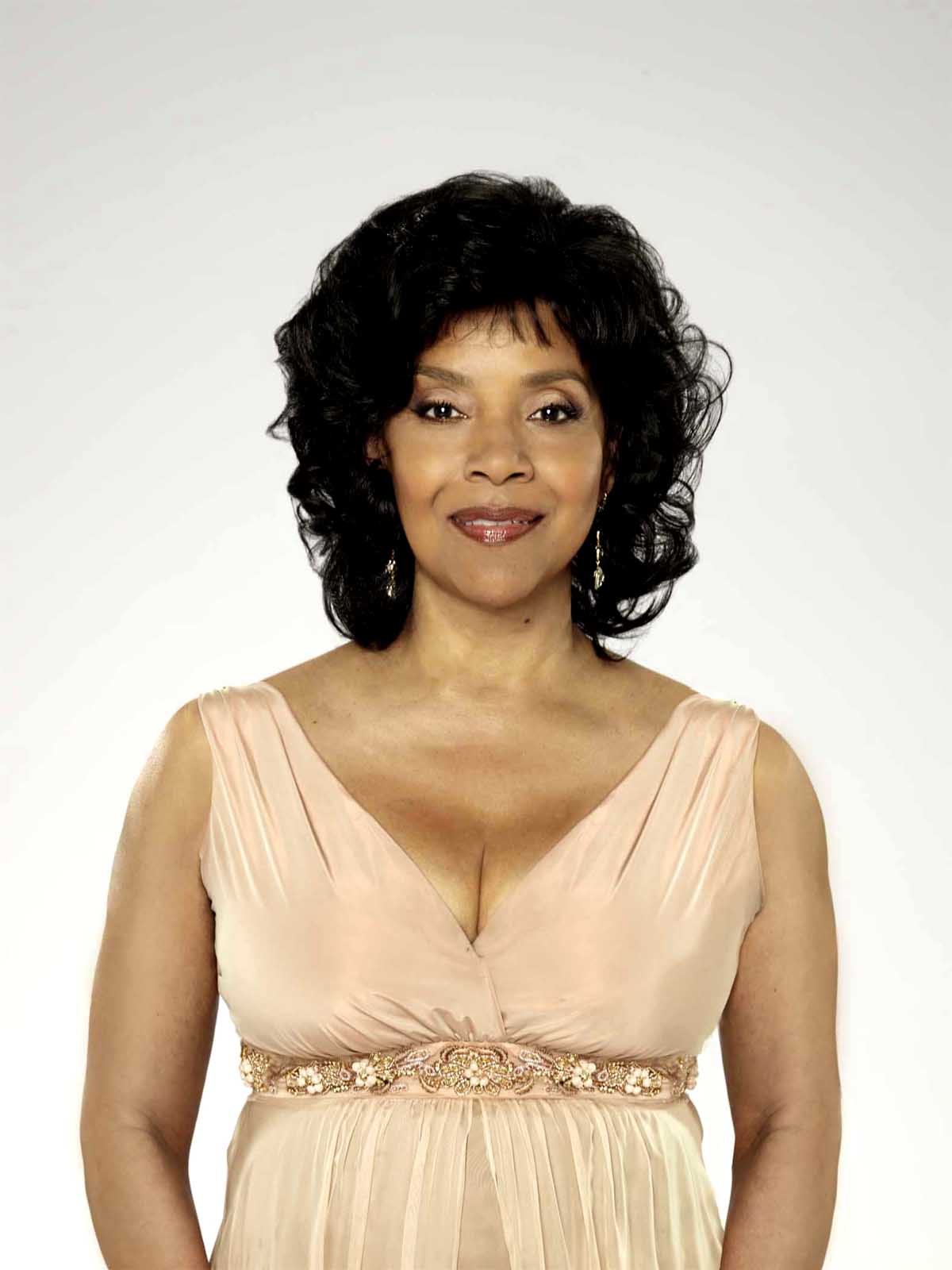This image features Phylicia Rashad, the renowned actress from *The Cosby Show*. She is standing and facing the camera with a gentle smile on her face. Rashad has voluminous, curly black hair that falls just above her shoulders. Her medium-brown skin is complemented by bold, red lipstick and subtle makeup enhancing her dark eyes. She wears a sleeveless, cream-colored dress with a touch of peach, detailed with a floral and beaded belt under her bust. Her gold earrings add a touch of elegance. The background is a gradient of light gray fading into white, providing a simple and clean contrast to her vibrant appearance. The photograph crops out just below her waist and at her arms, leaving her hands out of view.